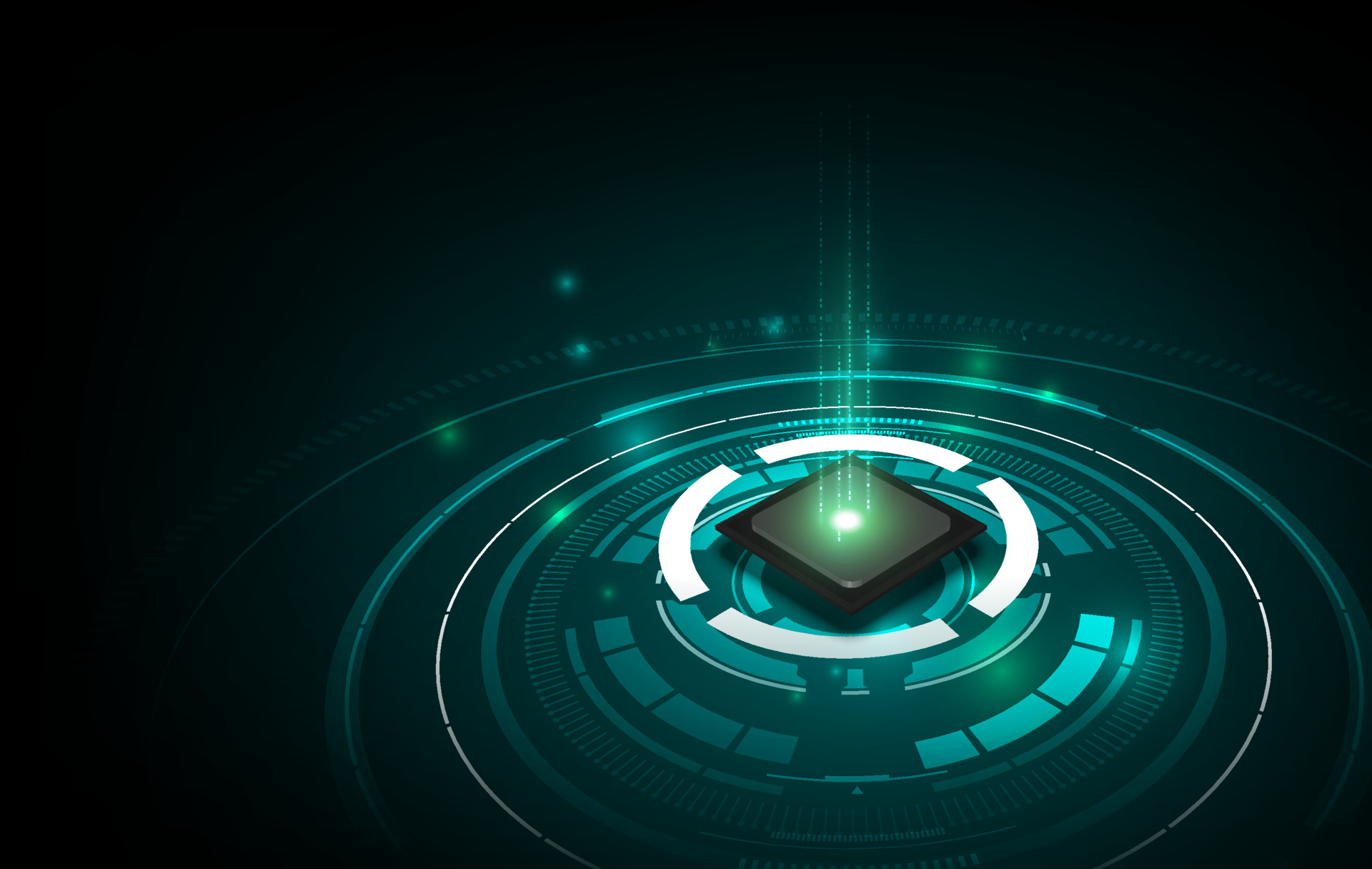The image is a detailed digital rendering, possibly used as a stock photo for technology or digital articles. The primary color palette features a striking green against a very dark black backdrop, creating a compelling contrast. In the bottom right corner, there are several concentric circular patterns of varying designs and colors—mostly green, but also with white and turquoise elements. The circles exhibit a variety of shapes including solid rings, rings with small rectangles, and rings with a mix of rectangle and square shapes. 

At the center of these circles sits a white sphere containing a black-outlined diamond shape with a bright green interior. Within this green area, a globe-like shape shines vividly, emanating green light upwards. This globe appears almost like a futuristic or cartoonish depiction of a computer chip or a central processing unit (CPU), suggesting a high-tech theme. The concentric circles and the glowing central element give the image a dynamic, almost otherworldly quality, as if zooming into the inner workings of a sophisticated digital or mechanical system.